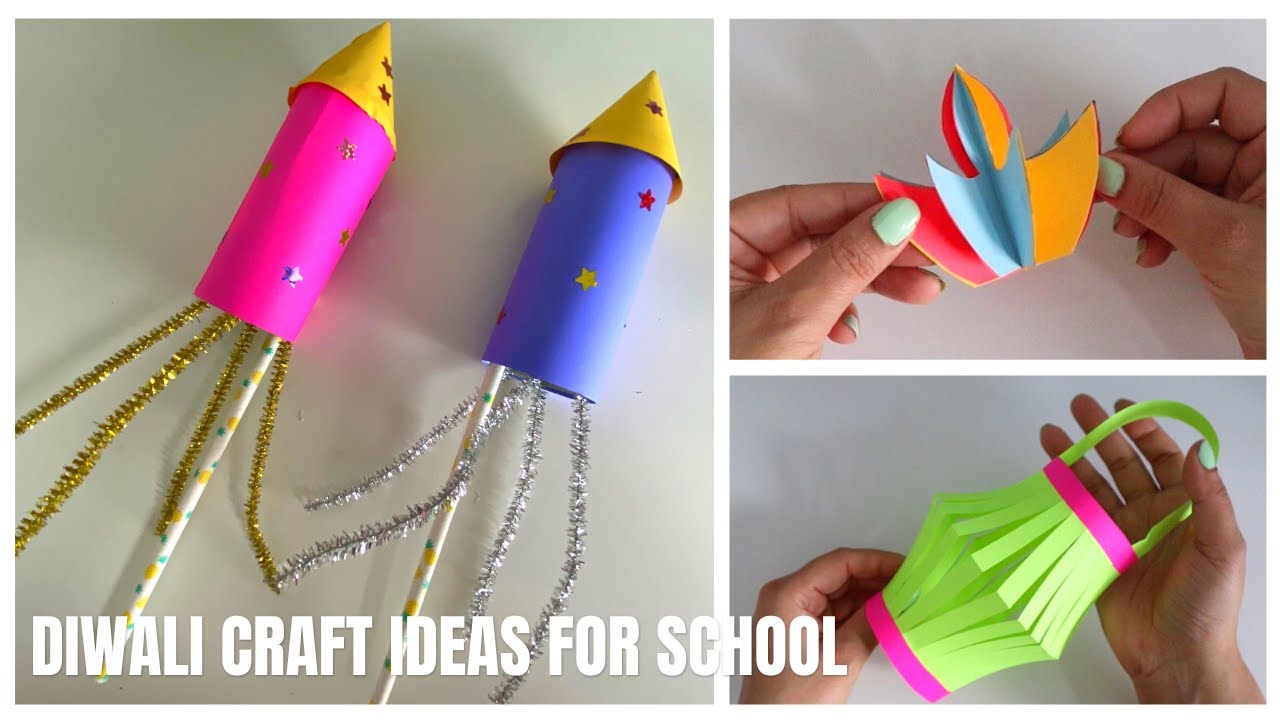The image is a collage featuring three separate photos showcasing Diwali craft ideas for school. The largest image displays two vibrant paper rockets made from brightly colored construction paper tubes, adorned with star stickers, and topped with golden and silver foil tails, attached to straws or pencils. The bottom of the image reads, "Diwali Craft Ideas for School." The top right photo depicts a spinning top crafted from folded blue, yellow, and red paper, resembling an intricate paper ornament. The bottom right photo shows hands creating an accordion lantern with lime green and pink paper, complete with loops at the bottom and a handle for hanging.